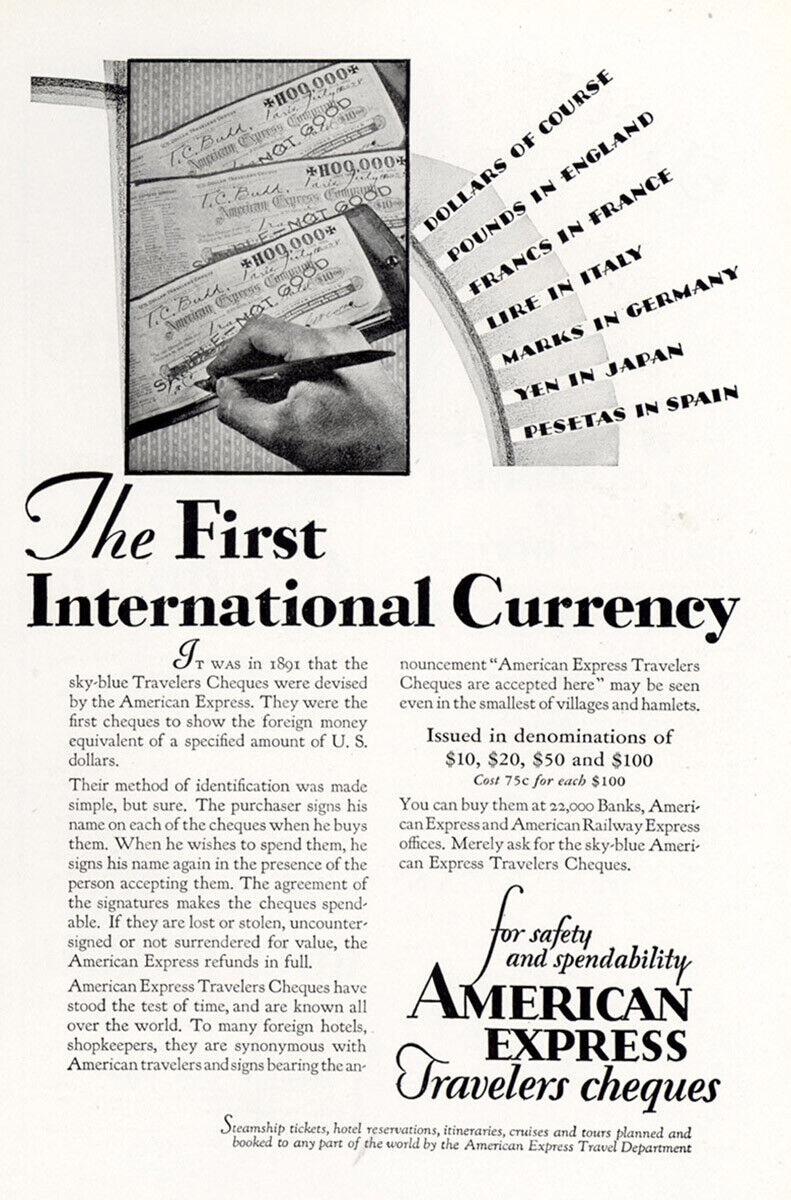The black-and-white photo appears to be a page from an old magazine, possibly slightly yellowed with age, showcasing an advertisement for American Express Traveler's Checks. In the upper left corner, there's an image of various international currencies, including dollars, pounds in England, francs in France, lire in Italy, marks in Germany, yen in Japan, and pesetas in Spain, with someone writing across them. The bolded text above the image reads, "Sample not good," indicating it's a sample copy. Below the image, a heading announces "The First International Currency," accompanied by paragraphs detailing that the checks are available in denominations of 10, 20, 50, and 100, costing 75 cents for each 100. The ad also emphasizes the availability of these checks at 22,000 banks. In the bottom right corner, it reinforces, "For safety and spendability, American Express Traveler's Checks," with the word "Checks" also styled in British English as "Cheques."